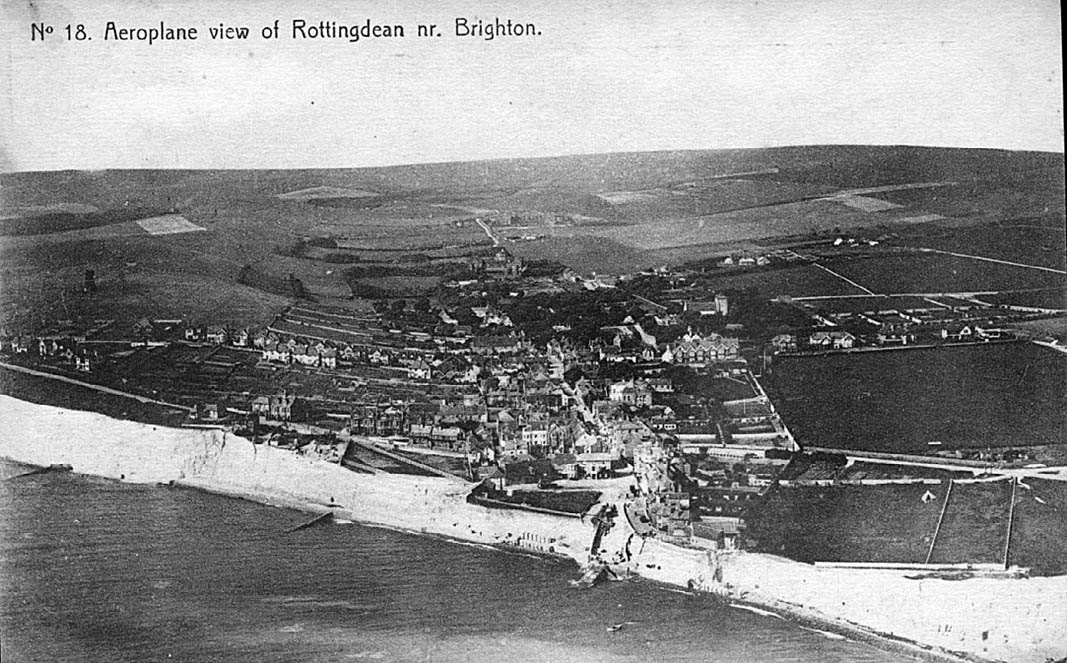This is a black-and-white, vintage aerial photograph of Rottingdean near Brighton, labeled "number 18 aeroplane view of Rottingdean near Brighton" in the top left corner. The photo, taken from an aeroplane, shows a bird's eye view of a coastal town situated along an extensive, white sandy shore that diagonally stretches from the center left to the bottom right of the image. The ocean occupies the bottom part of the photograph. The town appears nestled in a flat, gridded landscape dotted with buildings clustered towards the center, with large fields ready for agriculture surrounding it. As the view extends toward the outskirts, the scene becomes more barren with fewer buildings. The photograph is grainy and exhibits a slight rounding of the horizon about three-quarters up the image, giving way to the sky from that point to the top. The overall orientation of the image is landscape.